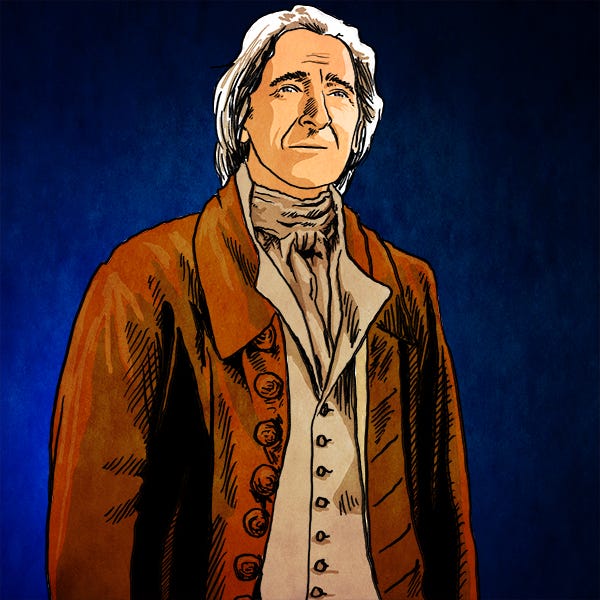This illustration features an older man, likely around 60 years old, portrayed in a cartoon-like style. He has white, somewhat long hair and no facial hair, accentuating his clean-shaven, wrinkled face. The man's attire reflects a colonial-era appearance, consisting of multiple layers: he wears a button-down vest in light cream with a neck scarf, all topped by a reddish-maroon coat with prominent buttons and a big collar. He stands against a bluish background, creating a stark contrast with his vivid clothing. The overall rendering is relatively simple and quick, using basic lines for shadows and textures, which suggests it may be from an animated series or comic book. The composition centers solely on this character, reinforcing his solitary presence in the illustration.